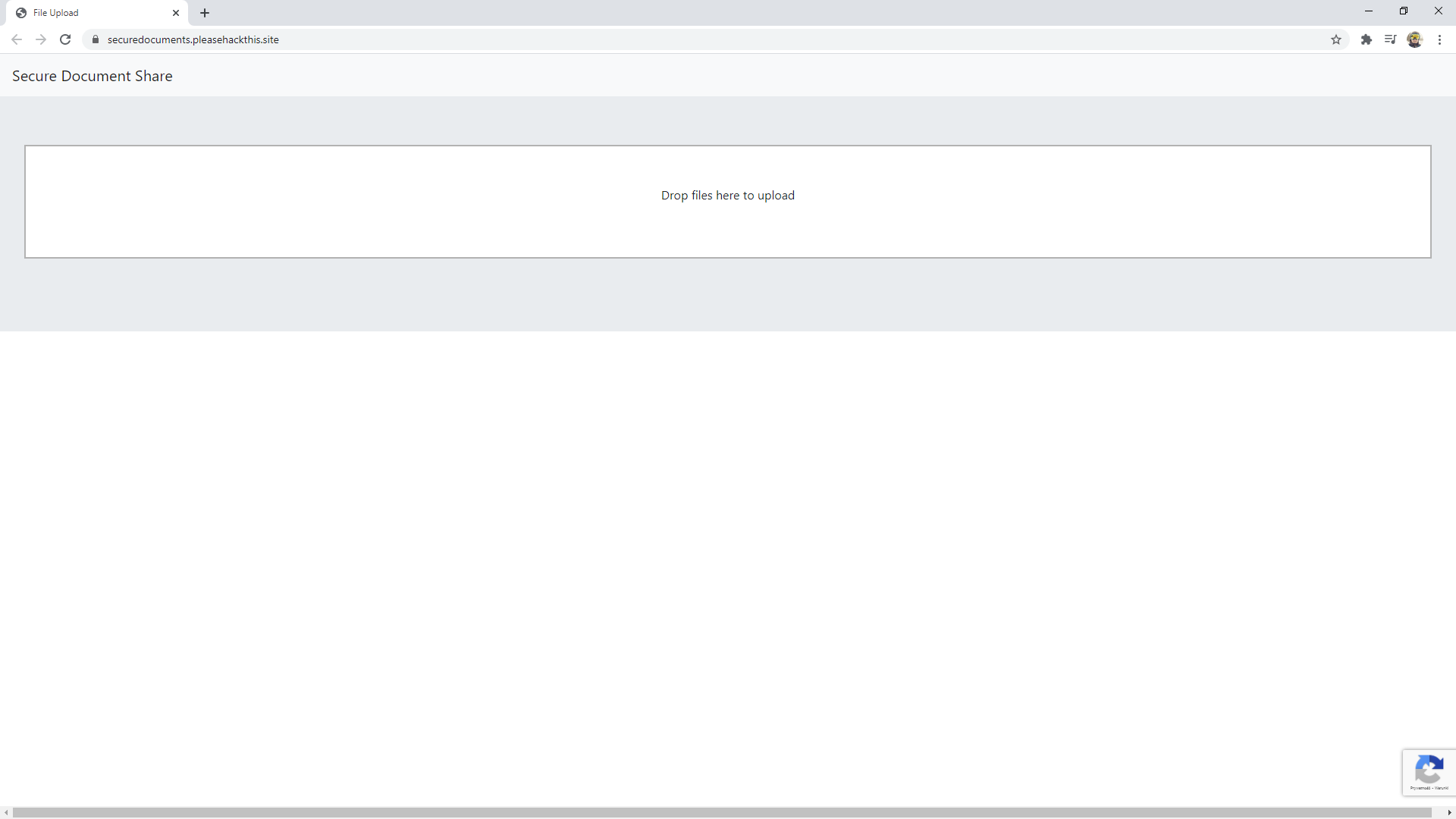The image showcases a browser window with various UI elements. At the top left, there is a white tab labeled "File, Upload" in gray letters. To the right of this is an 'X' button for closing the tab. Adjacent to this is a large gray tab with a black plus sign. On the far right, the interface includes a minimize line, a maximize double square, and a black 'X' for closing the window.

On the top left side, navigation arrows pointing left and right are visible, followed by a circular arrow which is the refresh button, and a search bar. Inside the search bar, there is a lock icon with the text "secured documents.pleasehackthis.site." To the far right of the search bar, there is a star icon, followed by a puzzle piece, a music note, and the user's sign-in picture.

Beneath the primary tab, the document is labeled "secured documents share" on the left-hand side. Below this, there is a light gray box with another white box underneath it. Inside the white box, the text "drop files here to upload" appears in gray letters. The rest of the box remains white. At the bottom of the main section, there is a large gray scroll bar that can be moved left or right, with arrows on either side.